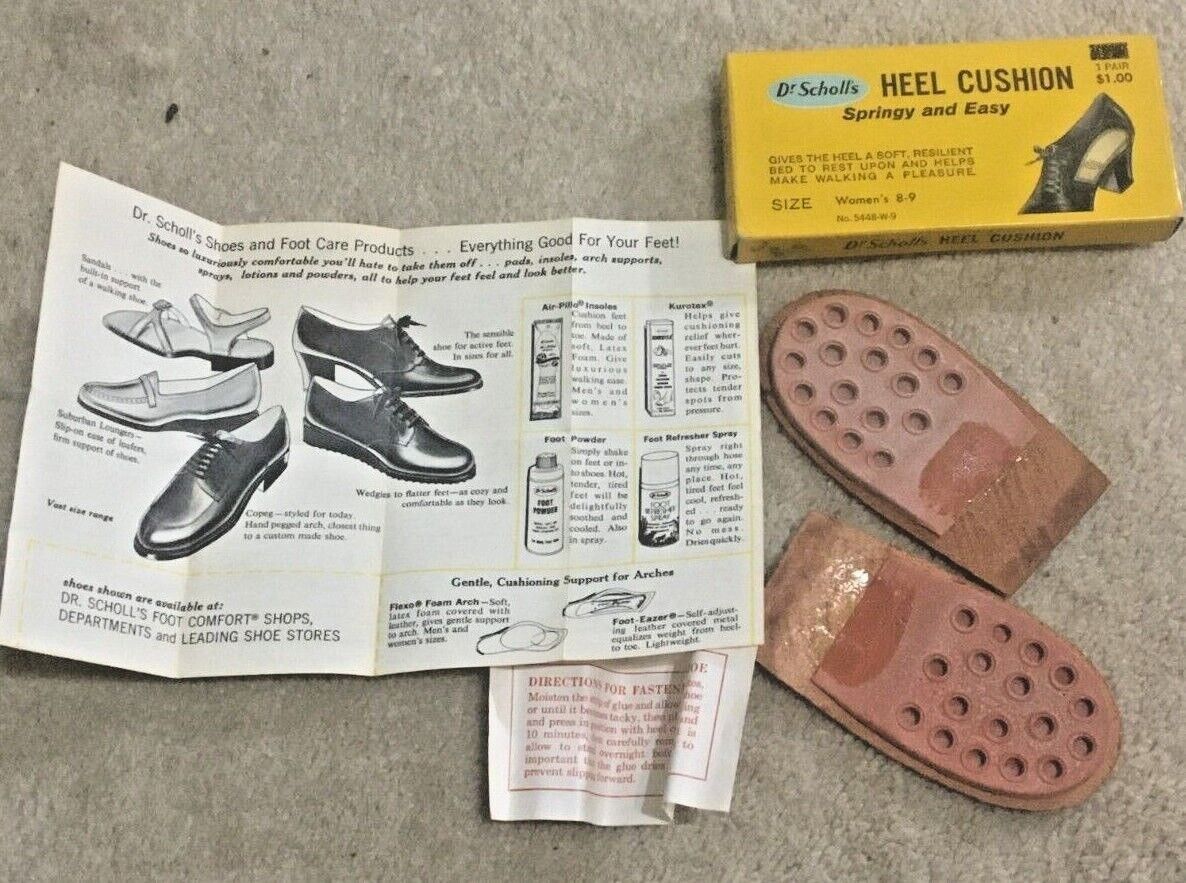The image shows a detailed top-down view of a pair of Dr. Scholl's heel cushions, set against a rough grey or beige rug. The heel cushions, which are pinkish-brown in color, are oval-shaped and have perforated bases designed for insertion into shoes. Positioned to the right side of the image, these cushions are stacked one above the other. A yellow box in the upper right corner reads "Dr. Scholl's Heel Cushion, springy and easy" in bold black letters, with additional text beneath. To the left side, there is a white manual or brochure that provides detailed instructions for using the heel cushions, including images of shoes and the inserts. The brochure features black text explaining the product's benefits and care instructions, stating phrases such as "gentle cushioning support" and "everything good for your feet." This setup provides a clear presentation geared towards fashion or footwear enthusiasts.